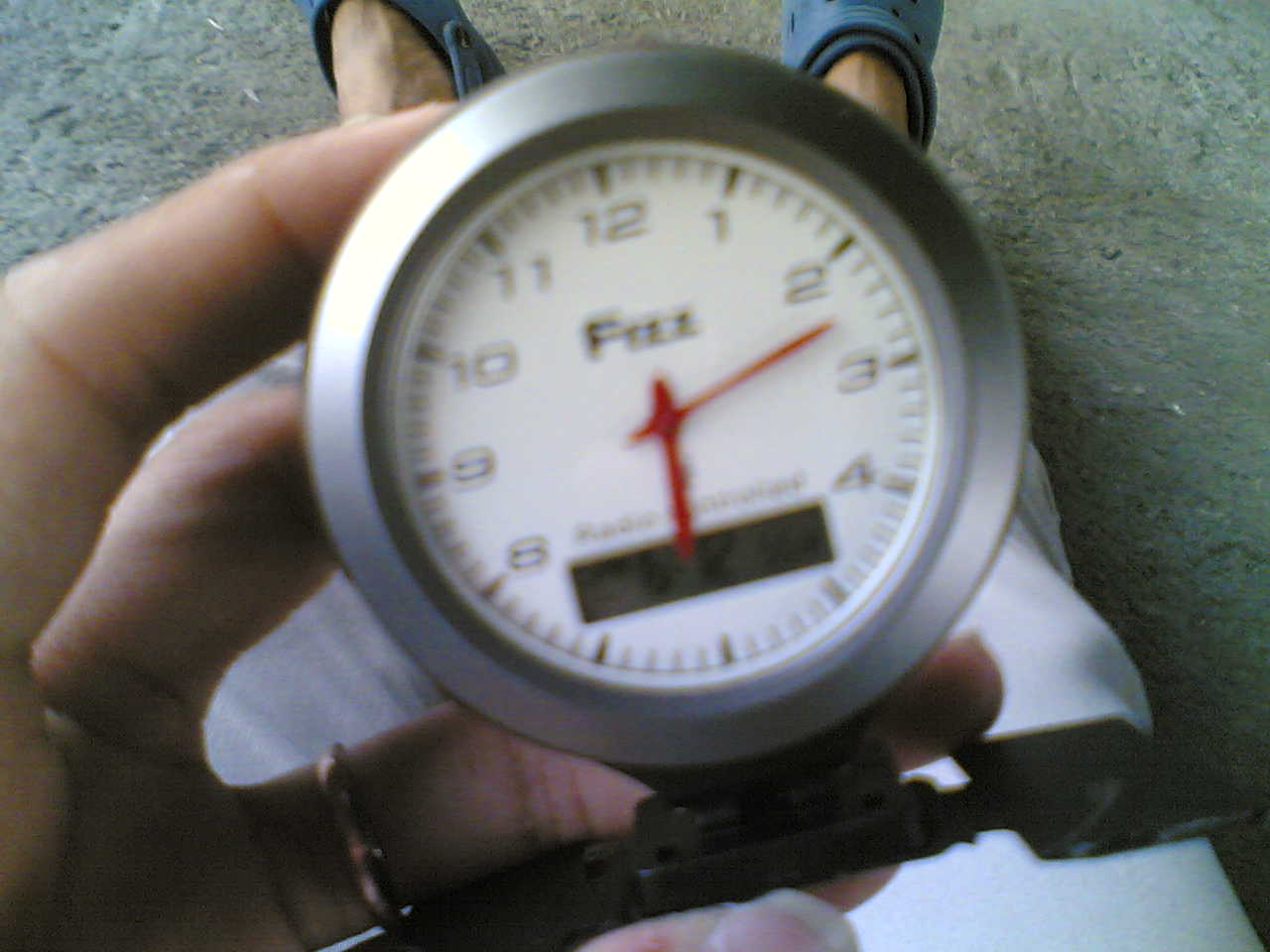In this close-up photograph, a person is holding a handheld clock, showcasing an intricate blend of analog and digital elements. The clock, made of brushed stainless steel, features black numbers 1 through 12 encircling its face. Below the analog display, a small digital screen offers a modern touch by also displaying the time. The person holding the clock is seated on a gray carpet, dressed in white pants and blue Crocs. Their hand, adorned with a gold wedding ring, gently grips the side of the clock. At the base of the clock, a small, flat metal mount is visible, adding to its functional design. The composition captures a serene moment, focusing on the detailed craftsmanship of the clock and the simplicity of the person's attire.